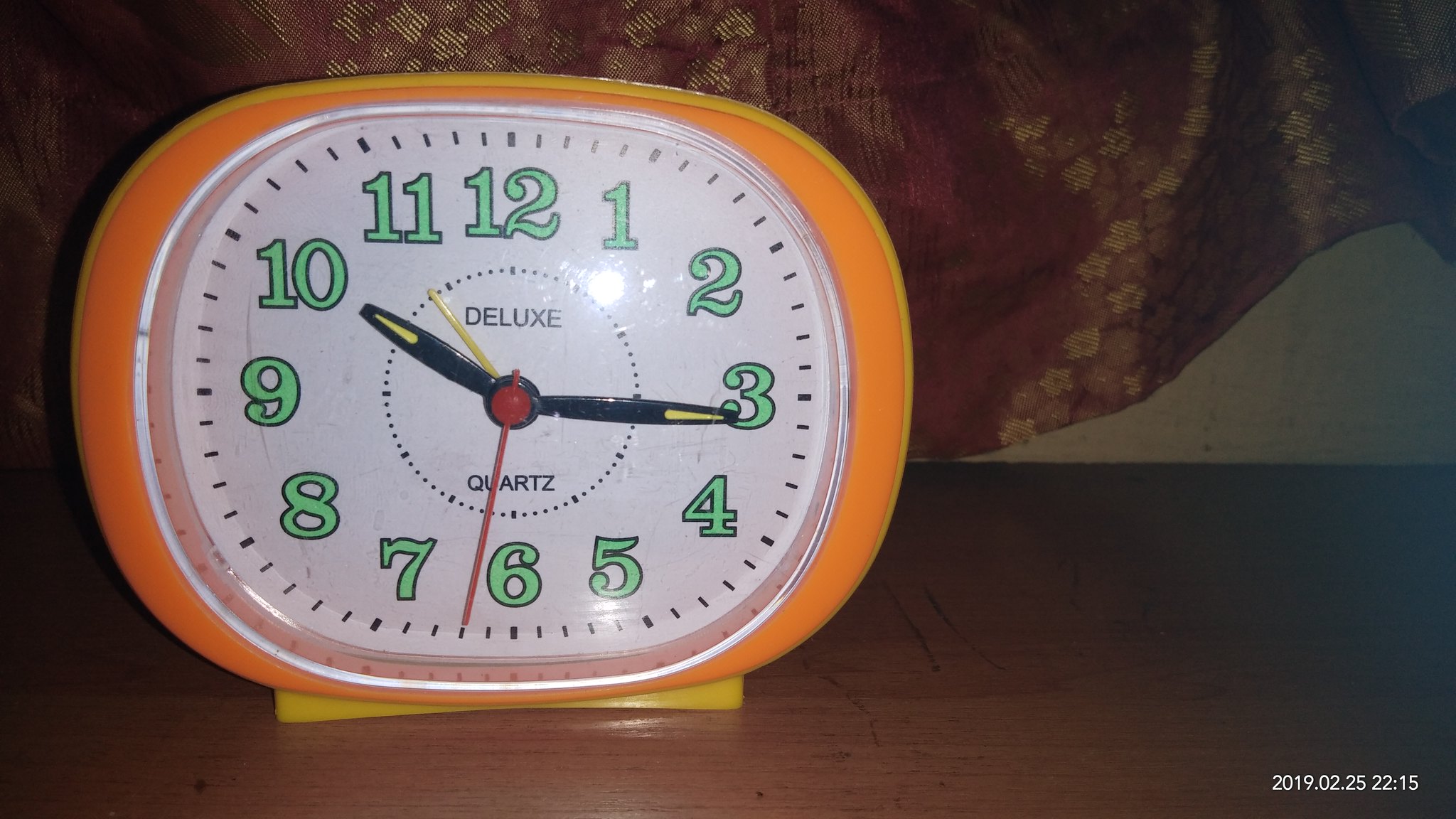This indoor, close-up color photograph captures a detailed view of a plastic, oval-shaped desk clock. The clock features an orange face encompassed by a yellow exterior and is supported by a small yellow stand on a light brown mantle. The clock's numbers are light green, and the black hour and minute hands are tipped with small yellow triangles. Additionally, a red second hand is positioned between the 6 and 7, while a yellow alarm set hand completes the timekeeping ensemble. The clock reads approximately 10:16. 

Central to the clock's face are bold black inscriptions, with "DELUXE" positioned above the dotted circle in the center and "QUARTZ" situated just beneath. Thick black dashes mark the hours, interspersed with thinner black lines for the minutes. In the lower right corner of the image, a time-date overlay states "2019.02.25 22:15."

The background reveals a cream-colored wall and a maroon-red curtain adorned with gold flowers, contributing to the richness of the scene. The photograph is taken in landscape orientation, accentuating the intricate details and textures of the desk clock and its surroundings.